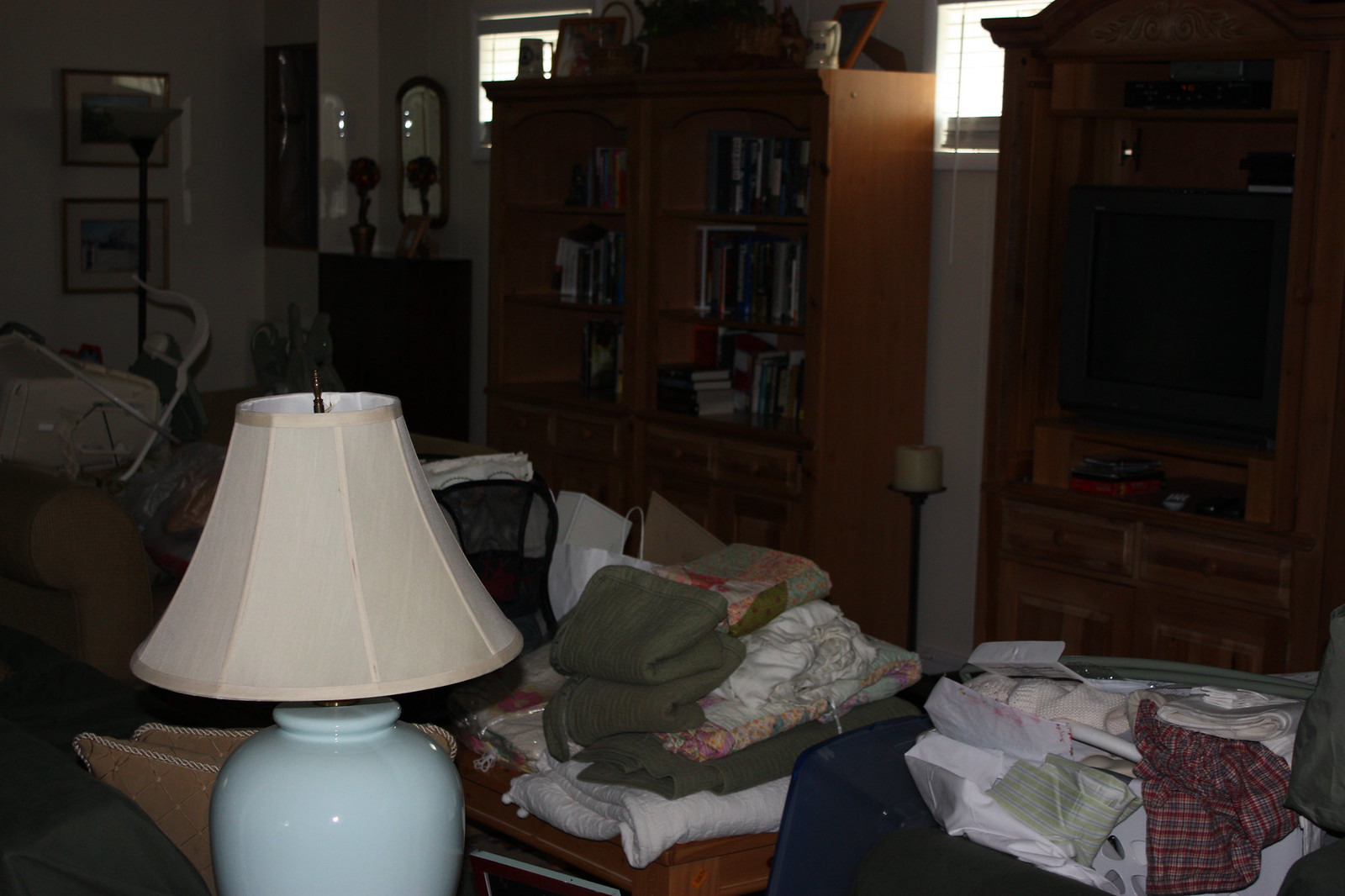A dimly lit room is depicted in this photograph, showcasing a cluttered yet intimate setting. In the foreground stands an elegant table lamp with a distinctive white, wide glass base. The base narrows at the bottom, widens towards the middle, and then tapers down before supporting a cream-colored lampshade that diffuses a soft, warm glow. Surrounding the lamp, a chaotic assortment of folded sheets, pillowcases, towels, and various other linens are haphazardly piled on a table, as if a linen closet has been hastily emptied.

In the background, wooden bookcases filled with an array of books line the walls, suggesting a well-lived-in space filled with stories and knowledge. A large metal candle holder with a candle approximately four inches in diameter adds a touch of vintage charm to the scene. Another cabinet, though not housing books, possibly serves as an entertainment unit, likely holding a TV or similar device. Despite the room's darkness, some natural light filters in through high windows, creating a faint but noticeable contrast to the otherwise dimly lit environment.